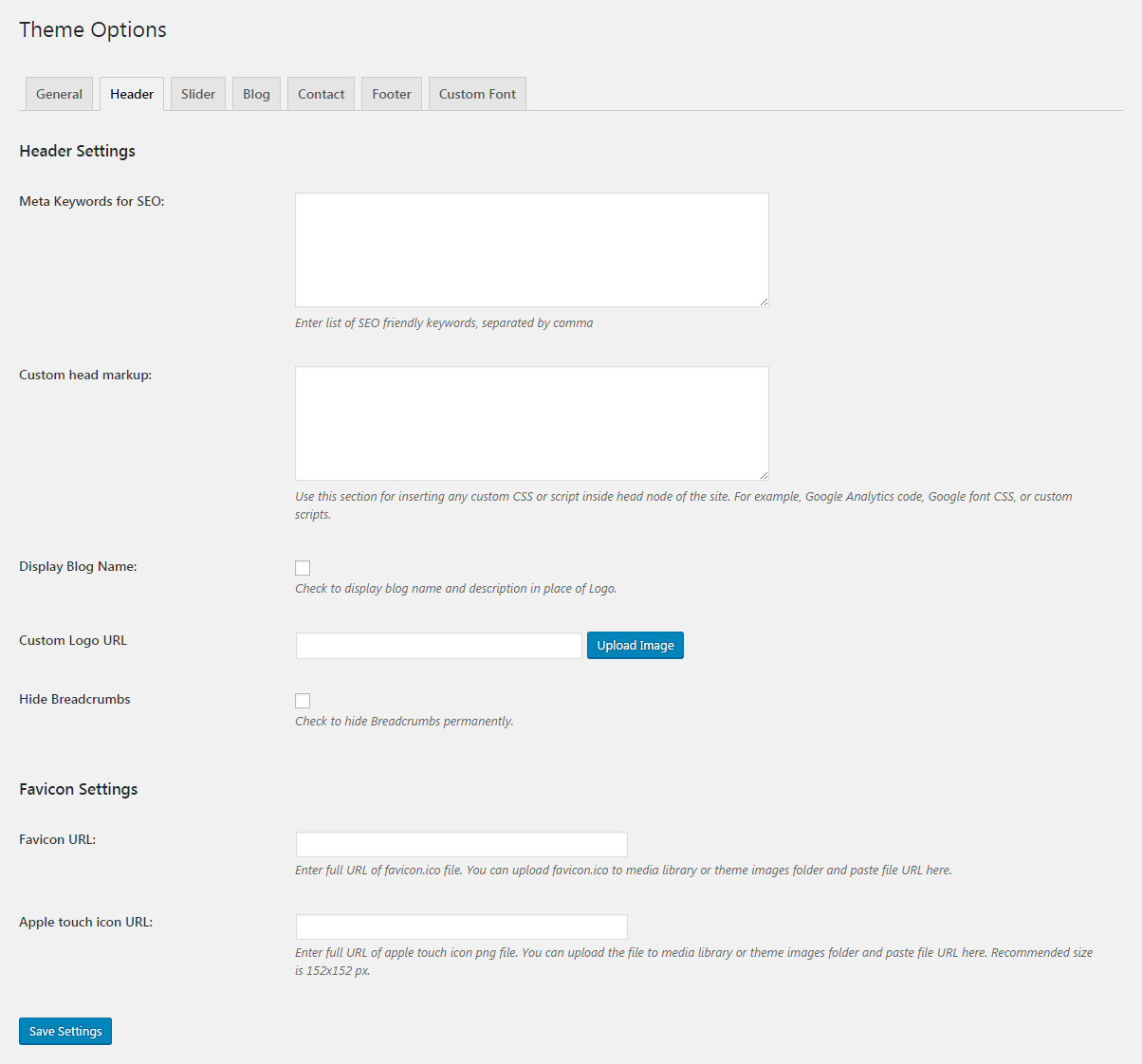This image showcases a webpage from a digital program or online platform, specifically displaying the "Theme Options" section. The background of the page is gray with predominantly black text, interspersed with some white and a small touch of blue.

At the top of the interface, there are various navigational tabs labeled as follows: "General," "Header," "Slider," "Blog," "Contact," "Footer," and "Custom Font." The "Header" tab is currently selected, revealing a set of related settings.

Below the "Header Settings" title, the first option is for "Meta Keywords for SEO," accompanied by an empty white text box where users can input a list of SEO-friendly keywords, with instructions to separate them by commas.

The next option, "Custom Head Markup," includes another writable box and a note encouraging the insertion of custom CSS or scripts within the head node of the site. Suggested uses include adding Google Analytics code, Google Font CSS, or other custom scripts.

Following this is the option to "Display Blog Name," which features a checkbox for activation. Another setting, "Custom Logo URL," provides an empty rectangular white box for input, alongside a blue "Upload Image" button for easy logo integration.

Additional options include "Hide Bread Crumbs," and fields for "Favicon URL" and "Apple Touch Icon URL." To finalize any changes, there's a prominent blue "Save Settings" button at the bottom of the section.